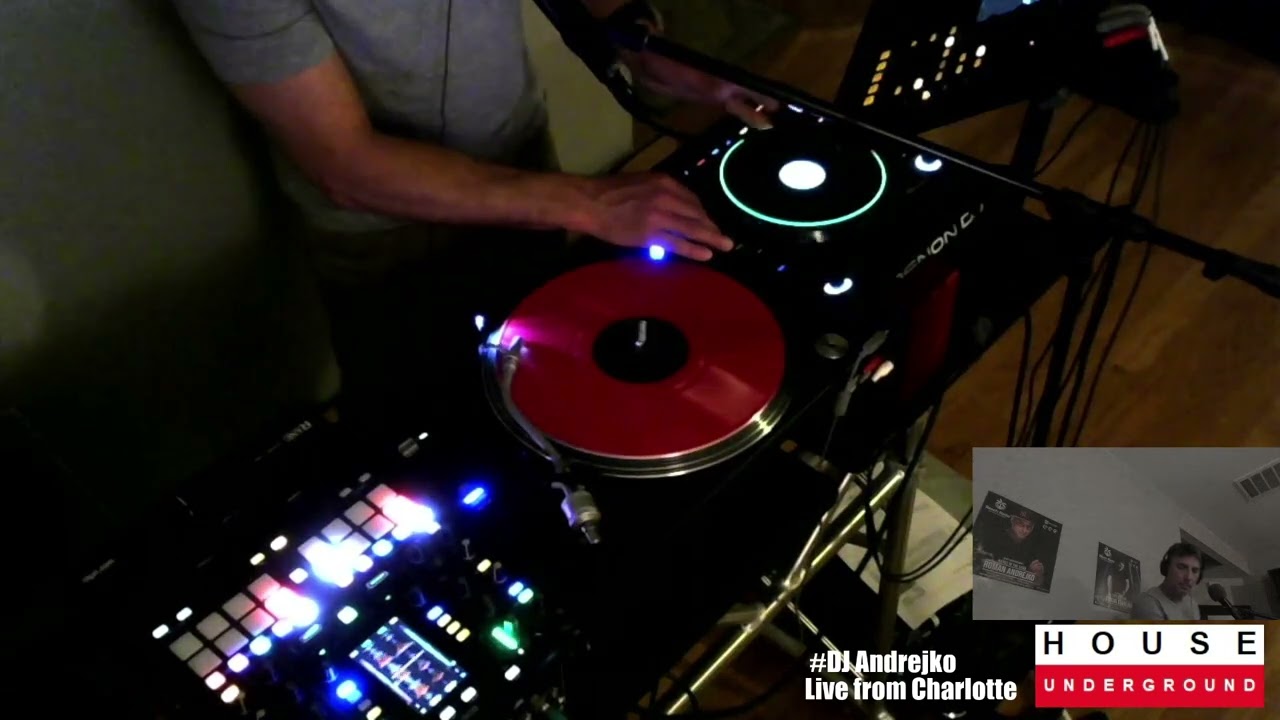The image features a muscular DJ, identified as DJ Andrzejko, performing live from Charlotte. He is seen wearing a short-sleeved blue button-down shirt and gray pants, with his arms stretched out as he manipulates a small black record on a dark turntable. His equipment includes a variety of controls and switches; to his left is a keyboard and a switchboard, while to his right, there is a larger red record on a turntable flanked by more lit-up controls of various colors. The scene prominently displays his DJ setup along with an insert showing his face. The logo "House Underground" and the text "#DJAndrzejko live from Charlotte" are visible, indicating that this might be a live stream screenshot or promotional ad.